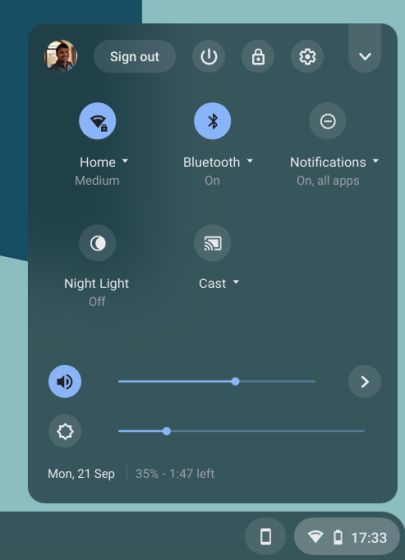The screenshot captured from a smartphone or tablet features a pale blue wallpaper adorned with a darker blue shape in the upper left-hand corner. The bottom of the screen is marked by a bar colored in a gray-green-blue hue. The header at the top of the screen displays oval-shaped icons for Wi-Fi, battery status, and the time, which reads 17:33.

Central to the screen is a prominent blue-gray rectangle with rounded corners. Inside the rectangle, the top left corner features a circular profile picture of a man in a button-up shirt standing in front of a window. Beside this profile picture are icons for signing out, a power button, a lock button, settings, and a drop-down menu indicated by a down arrow.

Below this section, there are several icons representing different statuses and functions. The first icon indicates that the device is connected to a Wi-Fi network named "home" with medium security. Subsequent icons show that Bluetooth is activated, notifications are enabled for all apps, nightlight is turned off, and TV cast is available. Further down, there are controls for volume and screen brightness adjustments.

At the bottom of the rectangle, additional information is displayed: the date, "Monday, 21 September", the battery percentage at 35%, and an estimated battery life of one hour and 47 minutes remaining.